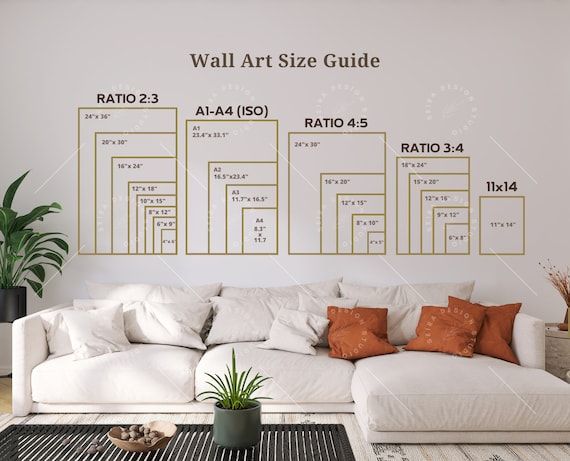The photograph captures a contemporary white living room featuring a sectional sofa backed up against a white wall. The sofa is adorned with a mix of white and red pillows, including a particularly long cushion on the far right. To the left of the sofa is a tropical leafy plant sitting in a black planter atop a light wooden table. In front of the sofa, there is a metal coffee table with slatted top, holding a giant circular steel planter and a small pink tray filled with stones. The entire scene is set on a white carpet. Dominating the back wall is a "Wall Art Size Guide" chart displayed in dark brown font, showing various size ratios and types of wall art, including ratios 2:3, 4:5, 3:4, and the smallest size of 11x14 inches, along with green-lined examples for each category.